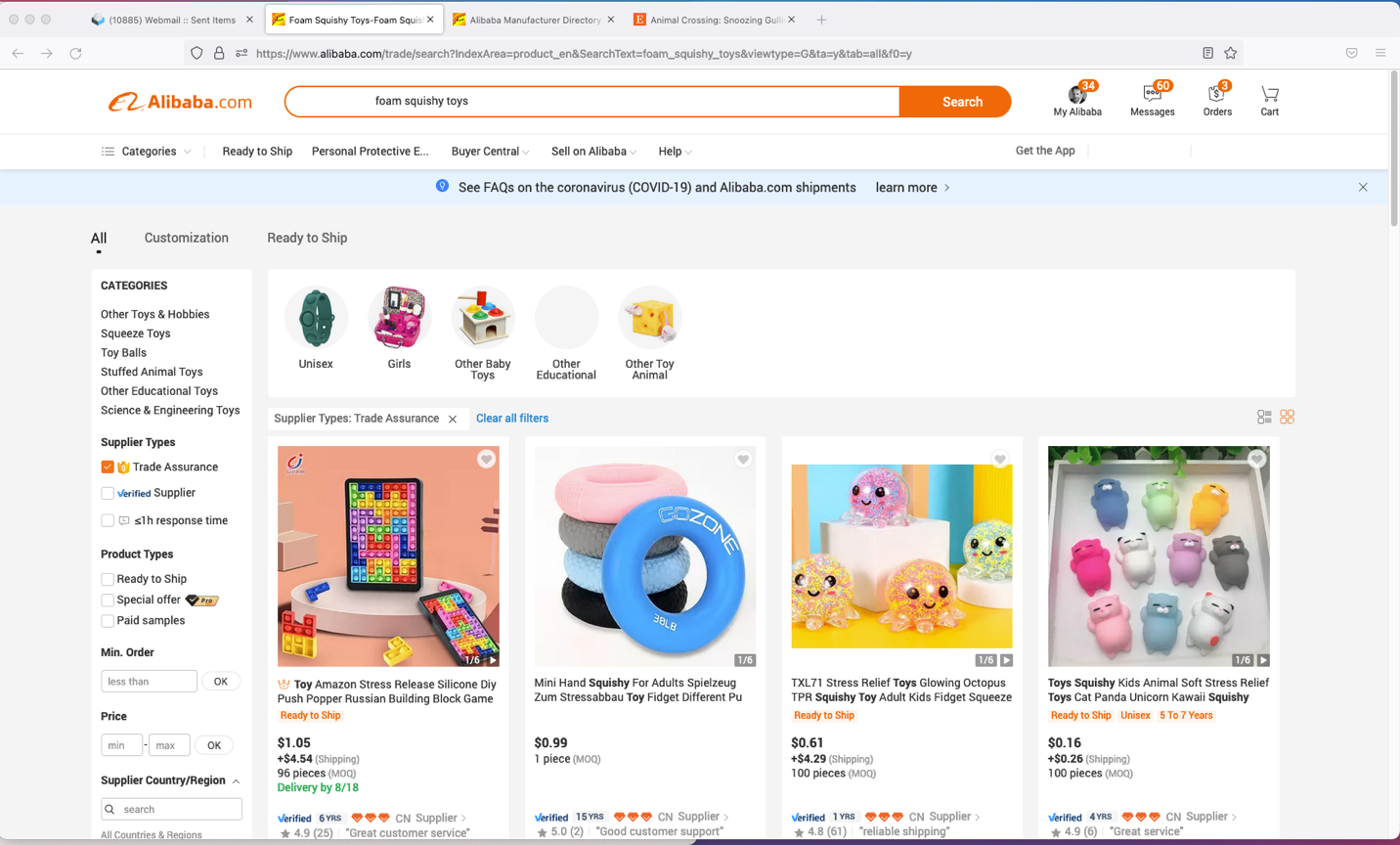The image depicts a website layout for Alibaba.com. In the top left corner, there are four browser icons, with the second one selected. Below the browser icons, the URL bar is visible. Next, in orange text, "Alibaba.com" is prominently displayed, adjacent to an orange search bar. The search field itself is white, with an orange search button on its right. Further to the right, four icons are presented. 

Beneath this section, six categories are listed in small black text, including options like "Categories" and "Help," with "Get the App" appearing towards the end. Additionally, there is a "FAQs" link directly below. 

The main content area is divided into sections, with category links running from top to bottom on the left. On the right side, five products labeled as "Ready to Ship" are displayed, all of which appear to be children's toys set against a white background. 

Further down, a larger image showcases four distinct products: a tablet on the far left, colorful pool floaties (in pink, gray, light blue, black, and blue) next to it, four stuffed octopuses, and finally, a collection of small animal toys for children. The overall background of the image is predominantly gray with significant white sections.